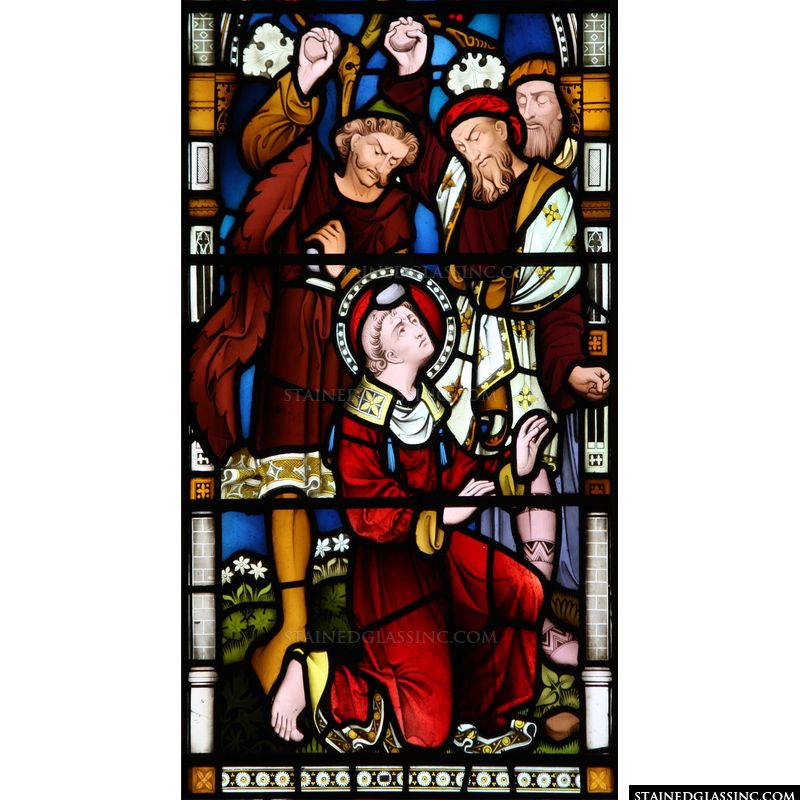This is a detailed stained glass window depicting a biblical scene. The window vividly portrays the stoning of a saint, who is identifiable by the halo around his head and his red gown. This saint is seen on his knees, raising his hands and gazing upward as he is pelted with stones. The colors used in the glass are vibrant, featuring blues, browns, golds, yellows, reds, and whites, all outlined in black. Above the saint, three men frown intensely, their eyes appearing closed or downwardcast, showing their determination to hurt him. The men are clad in various shades of red with different garments, including one with a golden-white vest. They all sport beards, mustaches, and some form of headwear. Each man holds a rock ready to be thrown. The scene captures a dramatic and somber moment, framed in three panes of glass, emphasizing its significance and sorrow. In the bottom right-hand corner outside the stained glass, the text "stainedglassink.com" is noted.